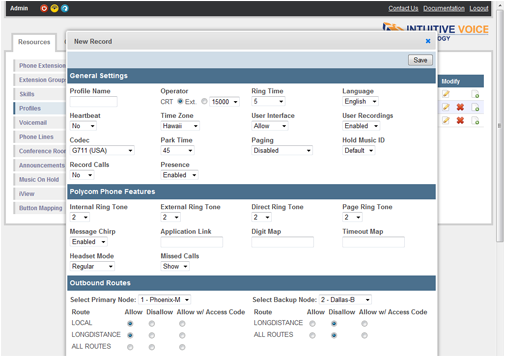In the upper left corner, there's an "Admin" label displayed prominently. Adjacent to it are three buttons: one red, one yellow, and one blue, all situated on a black bar that spans the top of the interface. On the right side of this bar are the options "Contact Us," "Documentation," and "Log Out," all in white text with an underline. Below these options, the text "Intuitive Voice" is visible.

A pop-up window overlays part of the screen, titled "New Record." Within this window, there are several labeled fields and drop-down menus: 

- "Profile Name" field, currently empty.
- "Heartbeat" with an empty drop-down.
- "Codec" set to "G711 (USA)" with a drop-down menu.
- "Protocols" labeled as "No" with a drop-down.
- "Operator" listed as "CRT."
- "EXT" is displayed in a blue circle.
- "15,000" within a drop-down menu.
- "Time Zone" set to "Hawaii" with a drop-down.
- "Park Time" set at "45" with a drop-down.
- "Presence" marked as "Enabled" with a drop-down.
- "Ring Time" with an unspecified drop-down menu.
- "User Interface" marked as "Allowed" with a drop-down.
- "Paging" marked as "Disabled" with a drop-down.